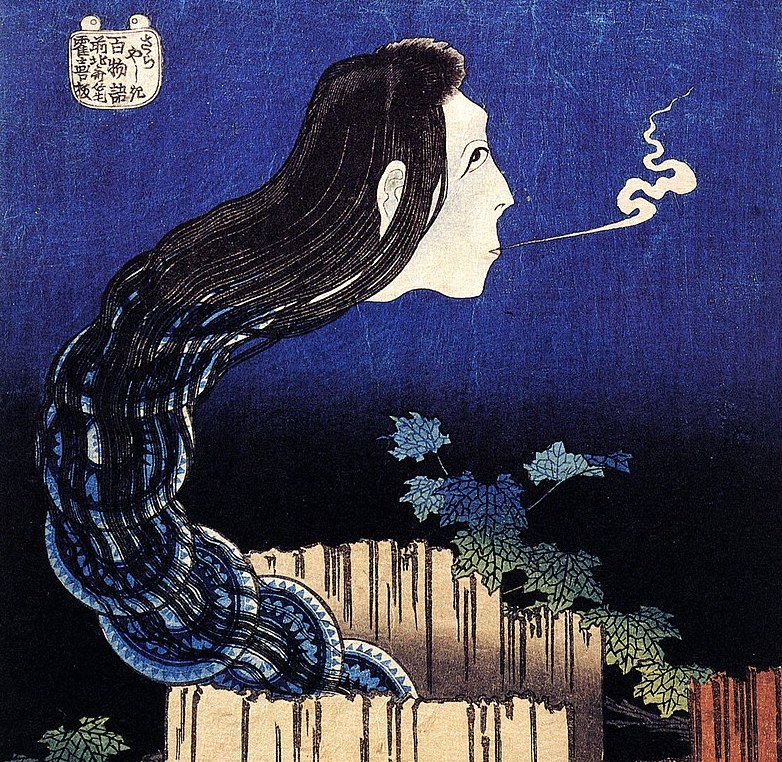The image depicts a striking and surreal illustration set against a gradient blue background that darkens to near-black at the bottom. A wooden fencing, light brown in color, wraps around itself in a loose horseshoe shape, with a darker section on the bottom right. Intertwined among the fencing are vine-like grape leaves, green at the bottom and transitioning to a reflective blue at the top. The left side of the fencing is adorned with a prominent green leaf.

Emerging from the center of the horseshoe-shaped fencing is a serpentine form, resembling a snake but composed of stacked circular segments that mimic blue and white plates. The snake-like body culminates in the head of a woman, her features indicating an Asian origin with long, flowing black hair cascading down her back. She exhales a cloud of smoke or hot breath, which trails to the left side of the image.

In the upper left corner, there is traditional Asian writing enclosed within a white shield, adding a cultural touch to the painting. The overall scene is reminiscent of Japanese woodblock art, with the character possibly representing a mythical naga—a creature with a snake's body and a woman's head.